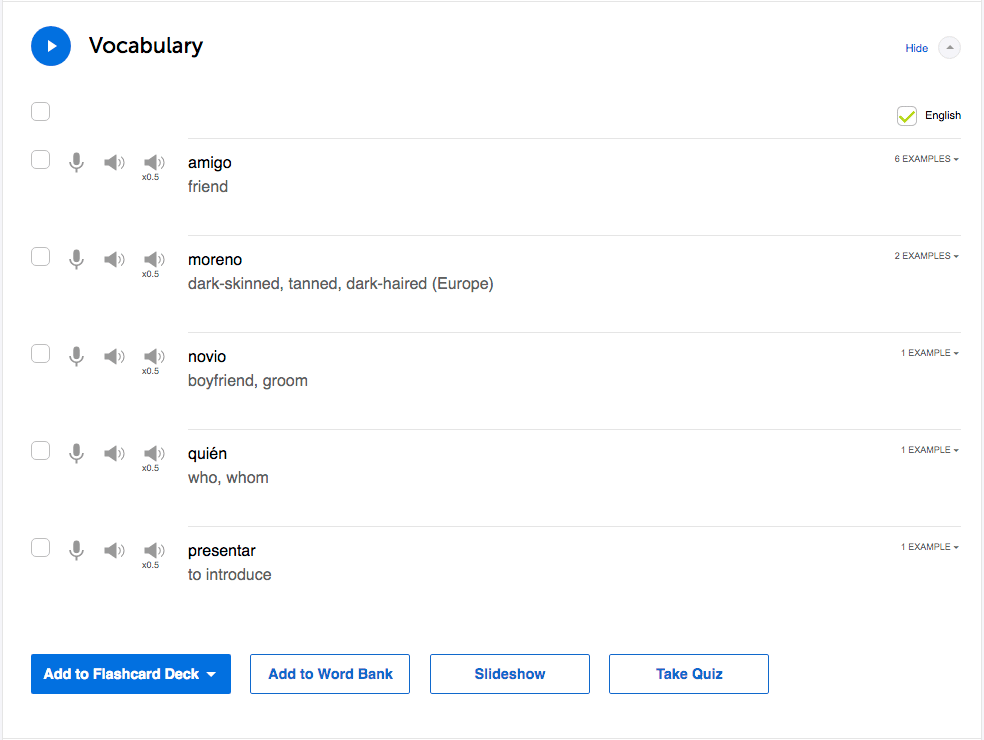A screenshot from a language learning app displays a dynamic interface dedicated to Spanish vocabulary. At the top center of the screen, a blue circle with a white play button is prominently featured, labeled "Vocabulary" in black text. In the upper-right corner, there's a "Hide" option with an adjacent toggle switch, though its specific function is unclear. Below this, a green checkmark indicates that the content is set to English. 

The main section lists several Spanish words alongside their English translations. "Amigo" is translated as "friend," "moreno" as "dark-skinned, tanned, dark-haired," "novio" as "boyfriend" or "groom," "quien" as "who" or "whom," and "presentar" as "to introduce." Examples using these words are visible on the right-hand side of the screen.

Users can engage with these words audibly, as there are options to play the pronunciations at varying volumes. At the bottom of the interface, several interactive options are available. A highlighted blue button on the left allows users to "Add to Flash Card Deck." Adjacent to this are white buttons offering functionalities such as "Add to Word Bank," "Slideshow," and "Take a Quiz." These features collectively create a robust tool for learning Spanish, indicative of a well-structured program.